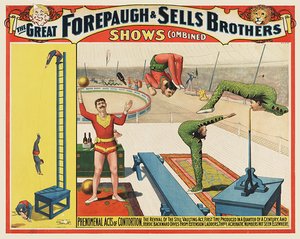This vintage circus poster from the 1920s or 1930s vividly advertises "The Great Fourpaw and Sells Brothers Shows Combined." Dominated by a red and yellow color scheme, the landscape-oriented artwork captures a bustling scene of various circus acts. The top of the poster features a prominent banner with the show's name, flanked by illustrations of a clown and a lion’s head. On the left side of the poster, a towering blue ladder supported by a wooden stand is the centerpiece; one performer is perched precariously at the top, leaning backward, while another is captured midair, hands outstretched, seemingly descending onto a platform, all dressed in blue unitards with red accents. Below them, another entertainer appears to be in the midst of a backflip. The right side of the poster highlights more acrobatic feats, with performers clad in leotards, contorting their bodies into dramatic shapes. Amidst them, one figure juggles a ball and a bottle, adding to the dynamic energy of the scene. The background features a circular area suggesting an audience ring, packed with spectators, emphasizing the lively atmosphere of the event.